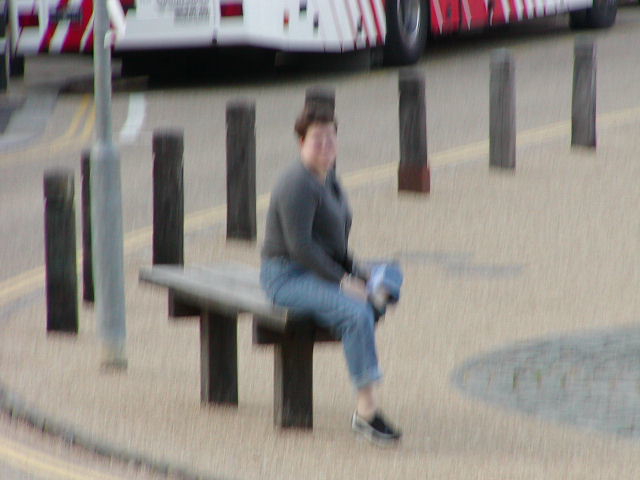A blurred image captures a woman sitting on a gray bench. She is clad in a gray pullover shirt and rolled-up jeans, with her feet sporting closed-toe slide shoes. Her attire and posture reflect a casual and comfortable demeanor. The woman sits with one leg propped up behind the other, creating a reversed number-four shape. She gazes toward the camera, her short, thick brown hair slightly tousled, and spectacles perched low on her nose, adding a thoughtful look as she peers over them. The background reveals a series of petite, decorative light projections arranged around the seating area, suggesting a cozy, well-lit environment. In the distance, a large vehicle, possibly a bus, is parked on the asphalt road, emphasizing the urban setting of the scene.